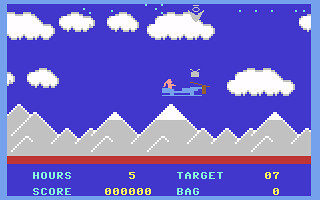The image is a detailed screenshot from an old video game, reminiscent of early Atari graphics. The screen is framed by a light blue border, with a dark blue background that fills the game screen. Dominating the scene are simple, triangular gray mountains with white lines outlining them, and some have white caps suggesting snow. Puffy white clouds dot the sky above the mountainous landscape.

In the sky, a light blue shape with a brown propeller-like element at the back and a pinkish shape that resembles a person is depicted flying. Near this flying craft, there is a gray, arrow-shaped indicator pointing downwards and a square, antenna-like gray object.

At the bottom of the screen, there is a red line, and below this line is a row of text displaying game metrics. The top row reads "HOURS 5" and "TARGET 87" in light blue text followed by yellow numbers. The bottom row shows "SCORE 000000" and "BAG 0," also in light blue text followed by yellow digits.